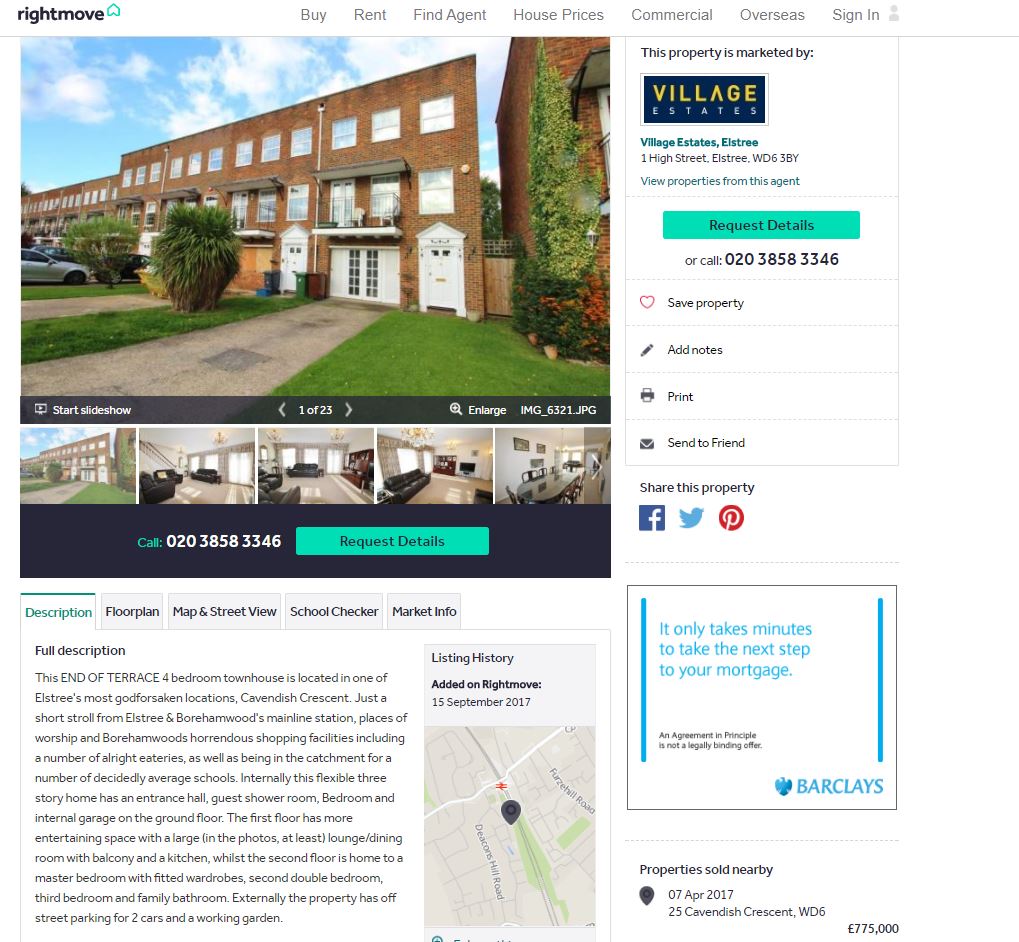The image displays the Rightmove website on a computer or another device, showcasing a property listing for an apartment. The platform specializes in real estate, featuring homes and apartments for sale or rent. The highlighted listing is for an apartment, identified as "Village Estates." A prominent image of a brick building is presented, accompanied by smaller interior photos. This particular listing includes a detailed description and a map tile indicating the approximate location, suggesting it is not within the U.S., as inferred from the international phone number. The interface provides various interactive options including a green "Request Details" button, along with features to save the property, send it to a friend, print the listing, add personal notes, or share it on social media platforms like Facebook, Instagram, and Pinterest.